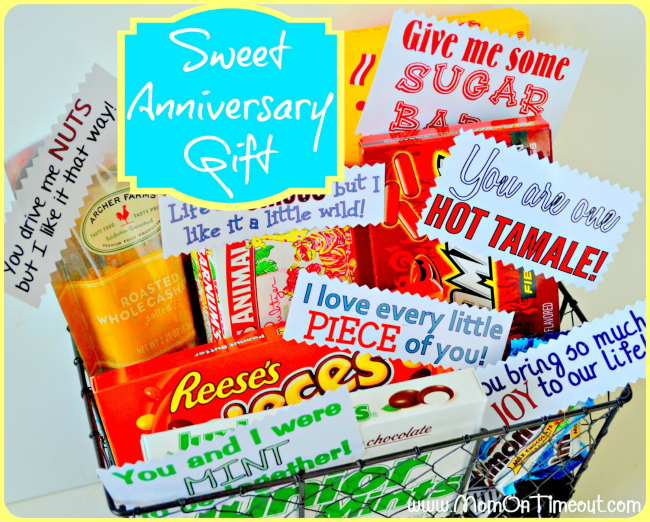The image features a black wire mesh basket, centrally positioned against a light blue background with a yellow border and white fonts, proclaiming "A Sweet Anniversary Gift." The basket overflows with various candies and snacks, each accompanied by playful, love-themed notes. Positioned prominently is a bag of Archer Farms roasted whole cashews with a note, "You drive me nuts, but I like it that way." Below are Reese's Pieces with the message, "I love every little piece of you." A small paper sign reading, "You and I were meant to be together," is affixed to a box of Junior Mints at the front of the basket. A box of Hot Tamales bears the note, "You are one hot tamale," while an Almond Joy says, "You bring so much joy to our life." At the top of the basket, "Give me some sugar, baby" graces a box of Sugar Babies. This clever, eye-catching advertisement combines the sweet and savory elements of anniversary love with a humorous twist.